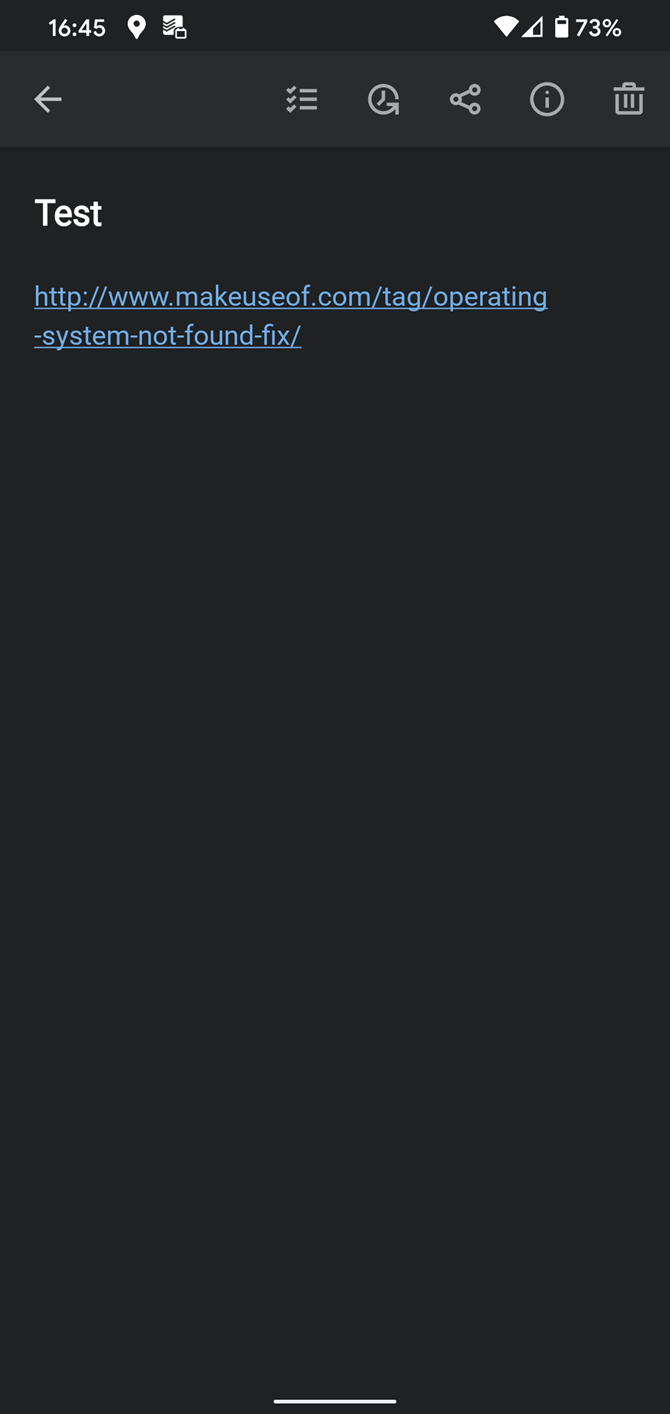The image shows a computer screen displaying a minimalist webpage. The background is completely black. At the very top of the screen, there is the word "Test" written in white letters. Just below this, a URL is presented in blue text: "http://www.makeuseof.com/tag/operating-system-not-found-fix/". This URL is underlined and clickable. 

The webpage extends downward into an unending black background. A thin white line is visible at the very bottom center of the screen.

In the system's status bar at the top right, the time reads 16:45. Next to the time, there is a white pin icon resembling a map marker, followed by an image icon, a blank area, and then the battery icon showing a 73% charge. The Wi-Fi indicator is visible, and there is also a small triangle icon. Additional clickable icons are located in the other areas of the status bar.